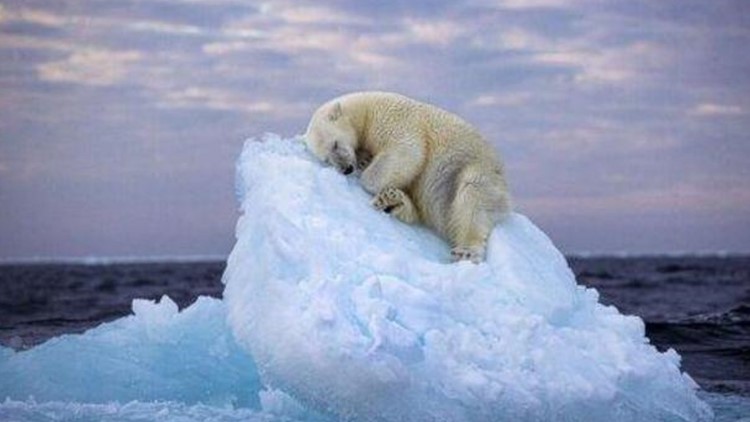This horizontal rectangular photograph captures a serene scene of a polar bear sleeping on a large chunk of ice floating in the ocean. The image, twice as wide as it is tall, centers on the bear, which is positioned facing the camera, with its head on the left and its rump on the right. The bear, with its thick, slightly off-white, yellowish fur, lies on its side in a semi-curled position on an angled block of snow-covered ice. Its front legs are crossed beneath its head, while its back legs brace against the ice to prevent it from sliding down. Surrounding the sleeping bear, the rough-textured ice appears choppy, perhaps melting, with a notable light blue piece of ice visible at the bottom left of the frame. The background features a dark navy blue ocean with choppy waters and a sky filled with pale blue hues along with gray and white clouds, suggesting a daytime setting. The overall focus remains on the tranquil polar bear, peacefully resting atop the angled ice floe amidst the stark, beautiful Arctic landscape.